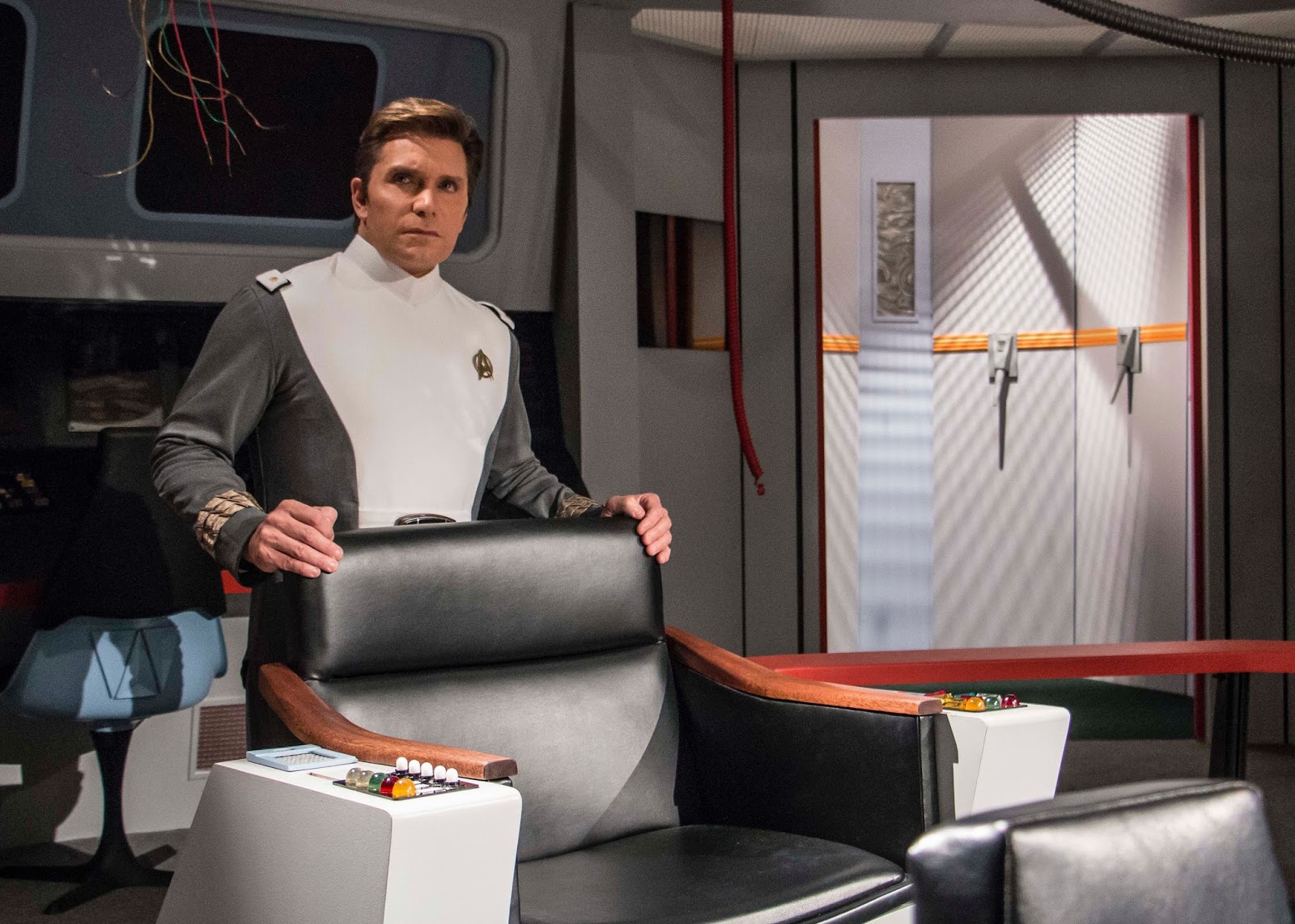The image appears to be set on a Star Trek spaceship set. In the foreground, there's a black leather chair with wooden armrests, each equipped with various control buttons and colored lights. Behind the chair stands a Caucasian man with medium-length dark brown hair, estimated to be around 40 years old. He is dressed in a futuristic gray and white Star Trek uniform, featuring a white torso and gray sleeves. The man is gazing slightly off to the side. The background reveals elements of a spaceship interior, including windows resembling part of a cabin, wires hanging from the ceiling, and a screen on the wall. To the right of the image, there is a section that resembles an elevator or a door, adorned with gray straps hanging on a yellow line. Additionally, a blue stool is visible, adding to the intricate details of the spaceship environment.